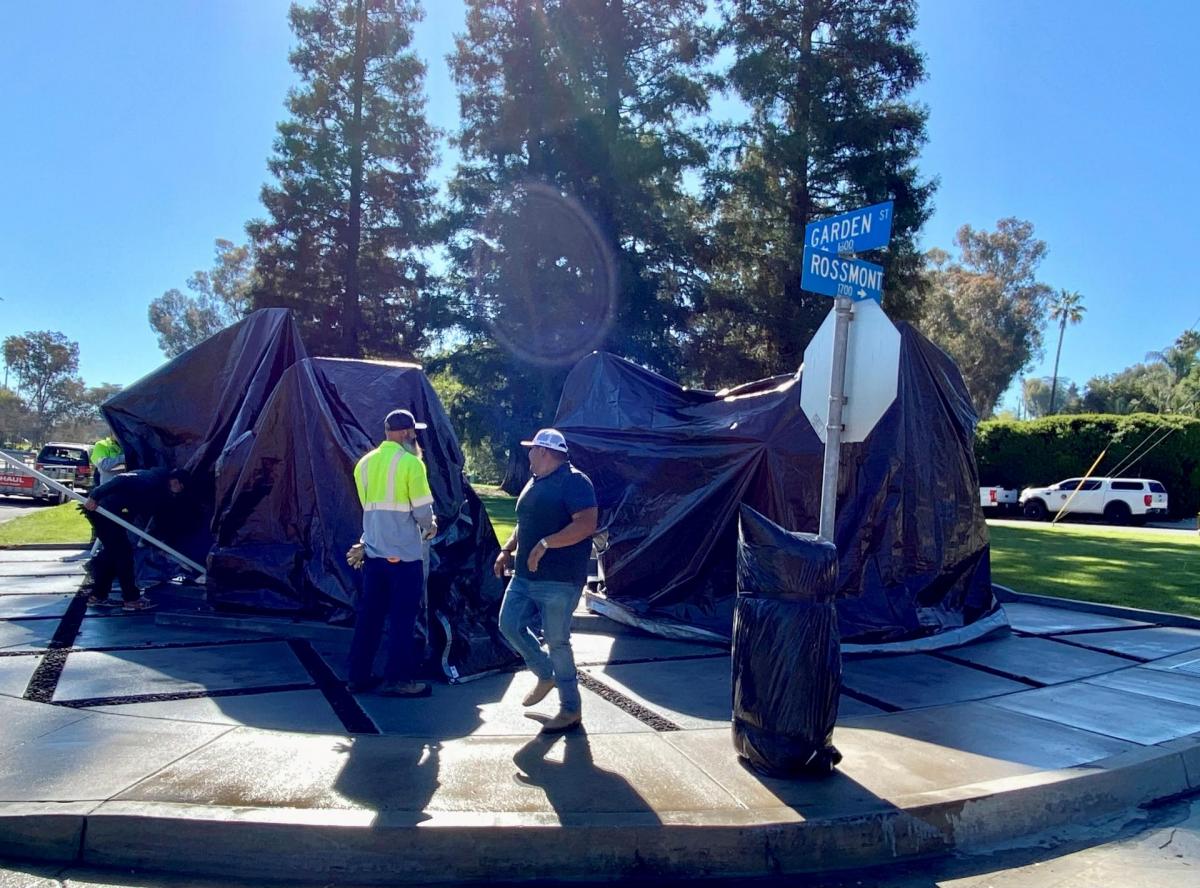This outdoor image showcases a landscaped corner at the intersection of Garden Street and Rossmont. Dominating the foreground are two street signs beneath a stop sign, set against a backdrop of tall trees and palm trees, suggesting a Californian locale. The scene is centered around a concrete pad that features a circular section with a sidewalk design, possibly containing asphalt markings. Several large, unidentified objects covered by black tarps are situated here, possibly hiding sculptures or machinery.

In the image, three to four individuals are engaged in activity related to these tarps. Noteworthy details include two men wearing baseball caps—one in a black shirt who appears to be conversing with another man donning a yellow safety vest. Additional workers are also visible, focusing on tasks near the tarps. Off in the distance, two white trucks and a van hitched to a U-Haul trailer are parked, highlighting the bustling environment. The overall impression is that of preparation, possibly for an unveiling event or a construction project.